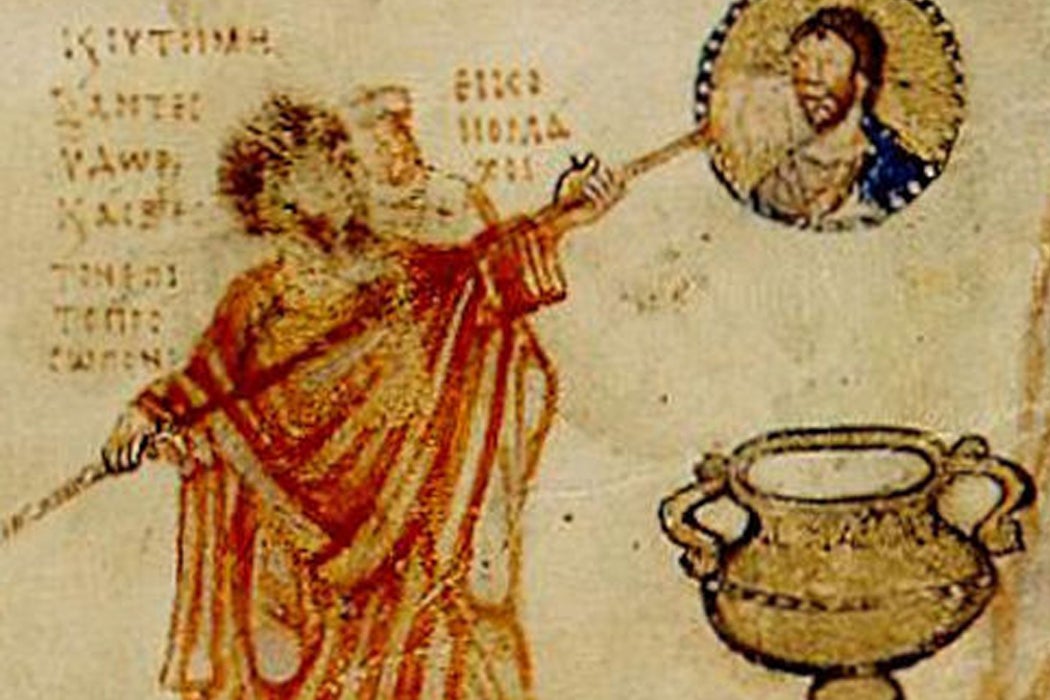The photograph captures a detailed scene from a religious painting rendered on parchment paper. In the top-left corner, there are seven vertical lines of writing, possibly in Latin, each line containing a single word. To the right of the text stands a figure clothed in a red robe, his face somewhat indiscernible. He holds aloft a long, golden staff with a circular end. Within this golden circle, there is an image of another man, depicted with brown hair, brown facial hair, and wearing a blue shirt, suggesting he is Caucasian with lighter skin. Beneath the staff and circle sits a large, ornate gold vase or cauldron. The entire page has a light yellow, slightly dingy beige background, enhancing the aged and historical essence of the illustration.